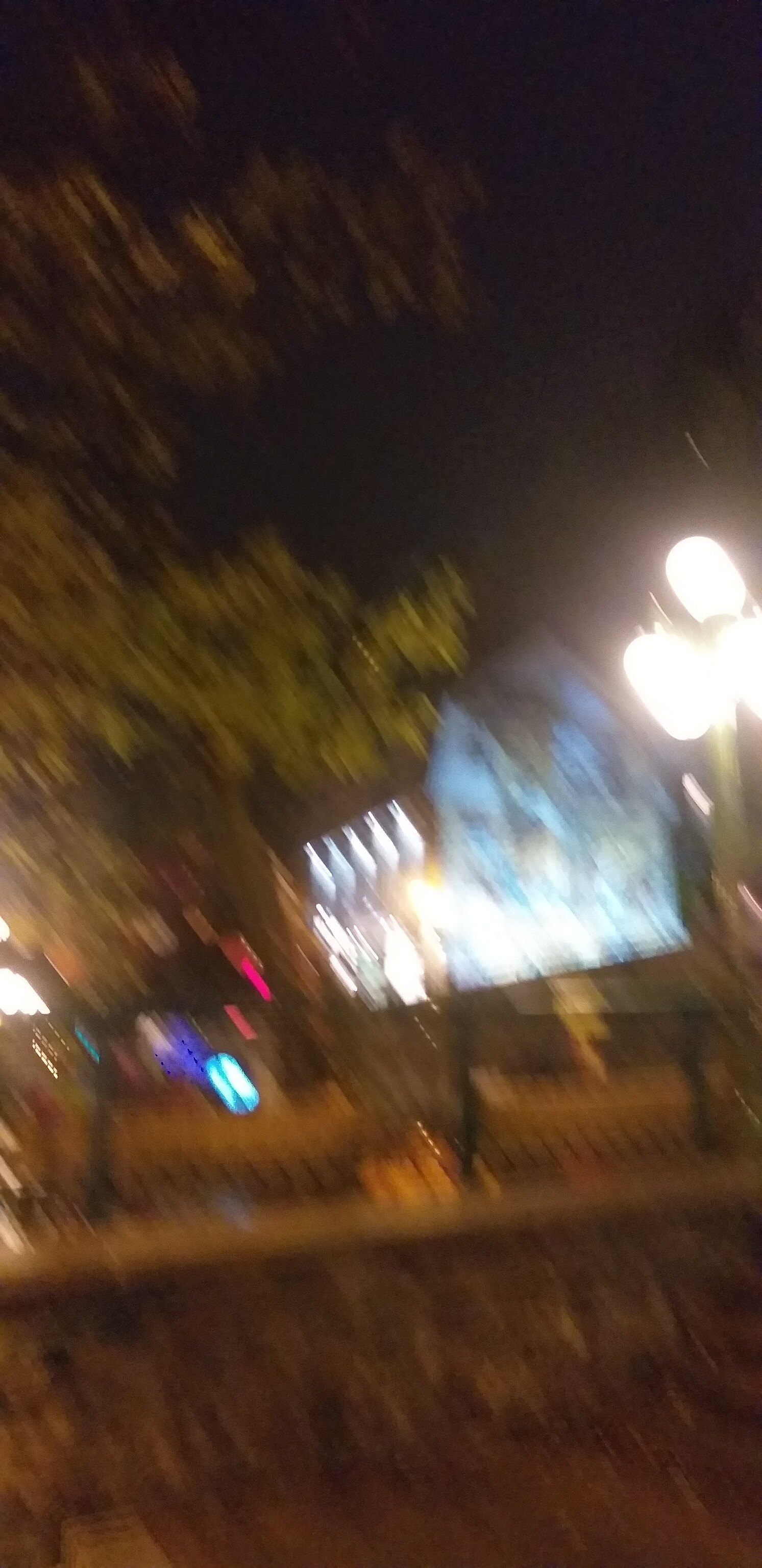A slightly blurry outdoor image captures a hilly landscape in the foreground, with a stone or concrete pathway running beneath a wooden park fence at the top of the hill. Behind the fence, several park benches are visible. To the left side of the image stands a prominent tree, while toward the center and right, street lights and the softly illuminated facade of a house come into view, casting a gentle glow on the surrounding area.